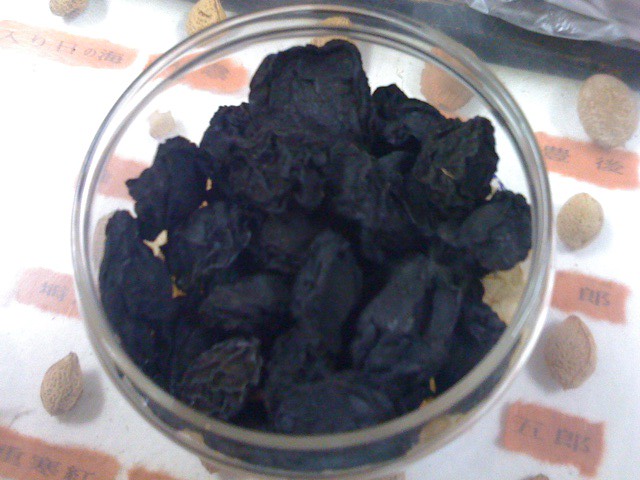The color photo depicts a detailed and organized display of various nuts, including what appears to be walnuts, almonds, and hazelnuts, arranged in neatly labeled rows on a white background. In the center of the image is a small, circular, clear glass bowl sitting on a clear glass countertop. The bowl contains about 20 dried blackish-blue fruits, likely raisins, which appear shriveled and bumpy, suggesting they are not in their freshest state. Each row of nuts beneath the glass countertop is separated by pieces of red-orange tape, labeled with writing that seems to be in Japanese or Chinese. The overall effect is a structured presentation, contrasting the varied textures and colors of the nuts and dried fruits with the clean, white background and clear glass elements.